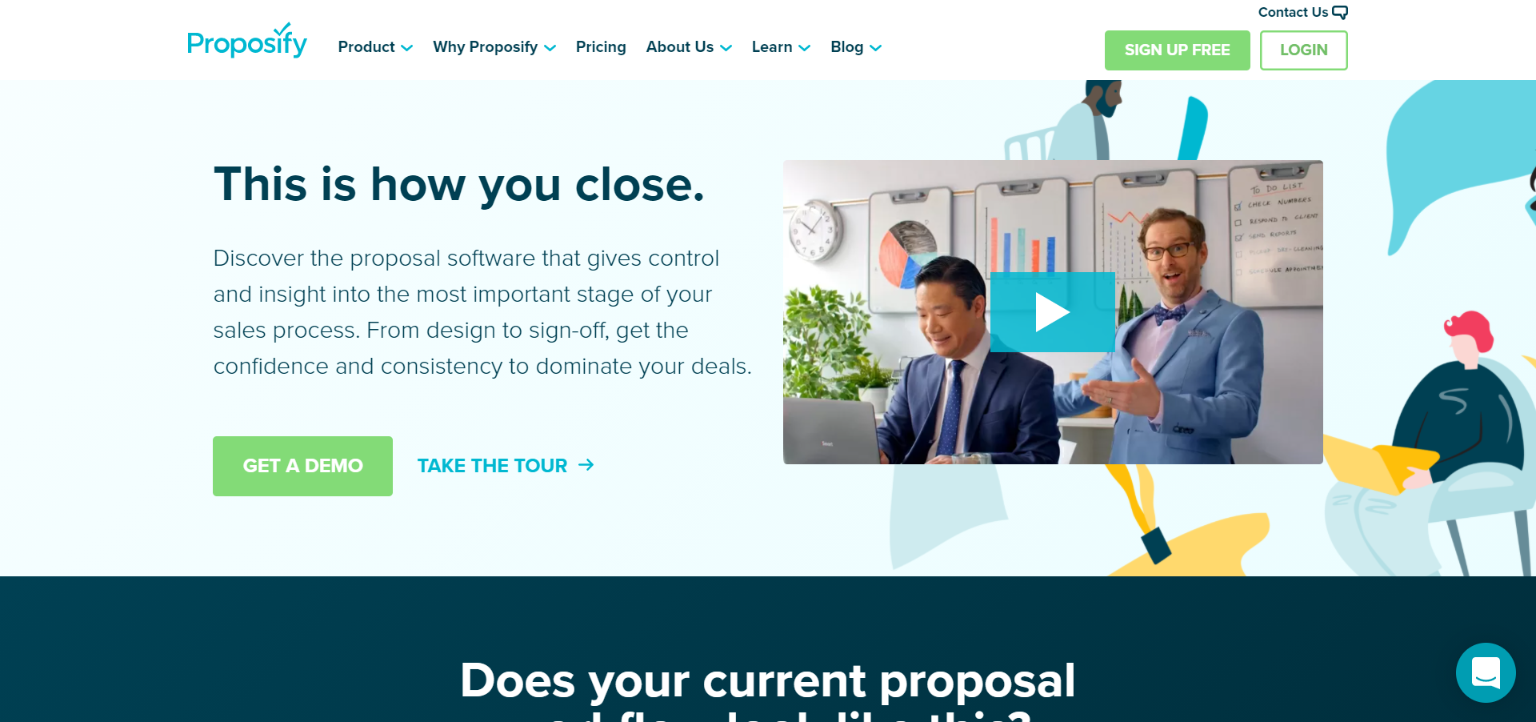This landing page from the company Proposify (P-R-O-P-O-S-I-F-Y) features a clean, engaging design. In the upper left-hand corner, the company's name stands out in bright blue text, with a distinctive blue checkmark replacing the dot over the 'i' in Proposify. To the right, a navigational menu in tiny navy blue text lists, from left to right: Product, Why Proposify, Pricing, About Us, Learn, and Blog. Further right, two prominent buttons catch attention: a green “Sign Up Free” button with white text and a white “Log In” button with green text and a matching green border. Above the Log In button, “Contact Us” is written in tiny navy blue text, next to a text icon.

Below the navigation bar, a horizontal rectangular section features a light blue background transitioning to an image of people sitting in various chairs, working on laptops. To the left on the light blue background, bold black text proclaims, “This Is How You Close.” Beneath it, a subheading reads: “Discover the proposal software that gives control and insight into the most important stage of your sales process. From Design to Sign-Off, get the confidence and consistency to dominate your deals.”

Underneath this text, a green box with white text invites users to “Get a Demo,” while a bright blue text link with a forward arrow encourages them to “Take the Tour.” Positioned on the right side, over the graphic of people with laptops, a small video player displays a still of two business executives: one seated at a table, looking at a laptop, while the other stands behind, looking excited.